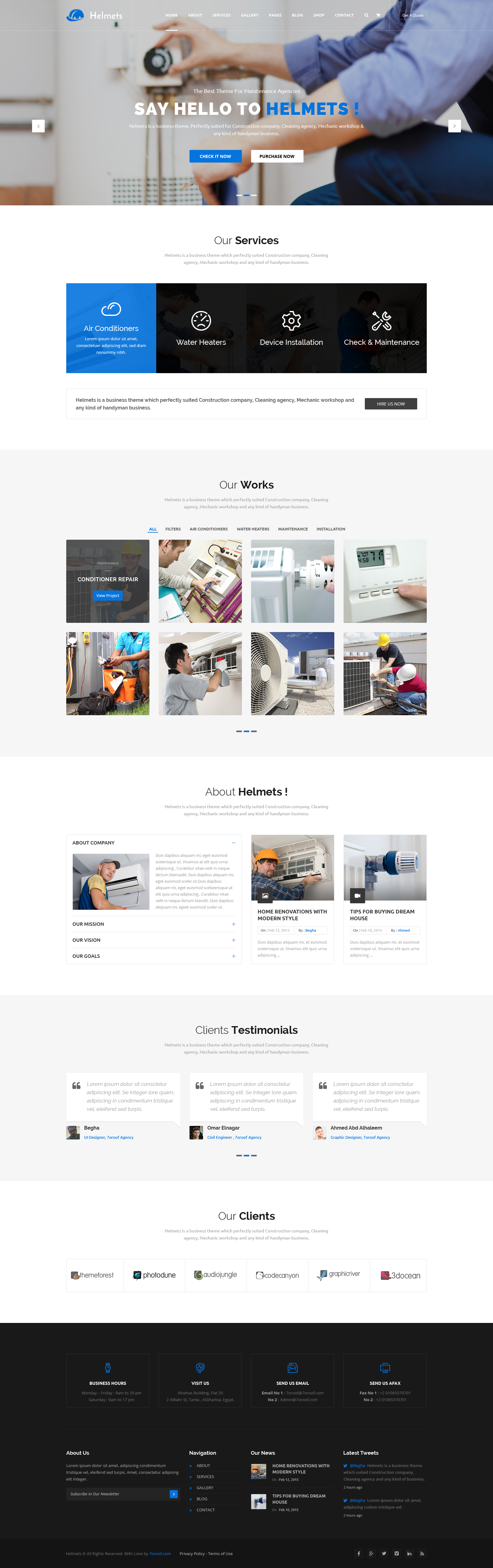A detailed caption for this image could be:

"At the top of the image, there is a person manipulating a dial on an unspecified device. Accompanying this are diminutive text and a symbol that are indistinguishable due to their size. Below this visual, bold text reads 'Say hello to' in white, followed by the word 'helmet' highlighted in blue. This text is set against a blue rectangle with a white rectangle beside it, each containing additional text. Beneath the main image, there's more text in black, accompanied by a blue rectangle housing a white symbol and text. Following this is a black rectangle displaying three distinct symbols, each with corresponding text underneath.

Further down, a pale gray rectangle features some text at the top, possibly a symbol, and additional text. Alongside this section are eight miniature images that are indiscernible. Adjacent to this is a white rectangle with text at the top, three small images, and text that are also too small to decipher. Below this, a light gray rectangle displays text at the top, along with three smaller white rectangles containing symbols and text, followed by an additional symbol and text underneath.

Finally, another white rectangle presents text and a series of symbols with adjacent text, leading to a black rectangle that has symbols at the top with text beneath them, followed by more text and additional, unclear symbols."